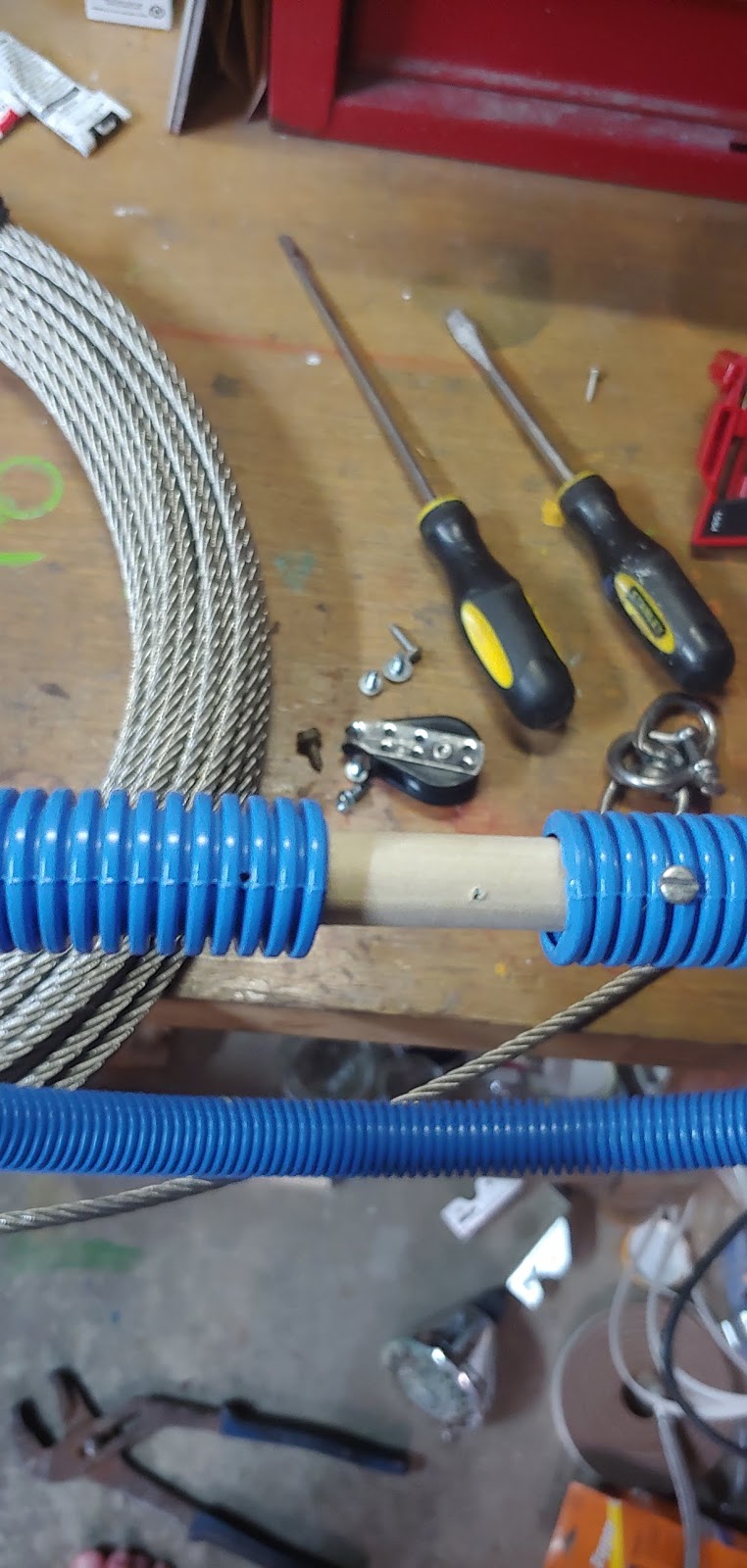In a well-organized woodworking and repair area, the image captures a detailed scene of a cluttered table in a garage, indicative of an ongoing project. The table itself holds a variety of tools, including both a flathead and a Phillips screwdriver, along with several screws scattered about. Evidently, someone has been disassembling items, as small metal parts are strewn across the surface. A coiled wire, meticulously wound into a circular shape, occupies much of the left side of the workspace, while a blue, seemingly stretchable tube adds a splash of color to the otherwise industrial palette.

On the concrete floor nearby, a wrench lies in plain sight, hinting at interrupted work or preparation for the next task. In the upper right-hand corner of the image, a red toolbox stands out, suggesting a well-stocked inventory of additional tools and supplies. The upper left-hand corner features tubes of what appears to be adhesive or glue, essential for various repair tasks. Closer to the bottom of the picture, a showerhead is casually placed on the concrete, adding a layer of curiosity about the project's nature. Additionally, an orange item, possibly a label or part of a packaging, is noticeable in the bottom right sector, adding another element to the array of utilitarian objects in this rich, detailed scene.